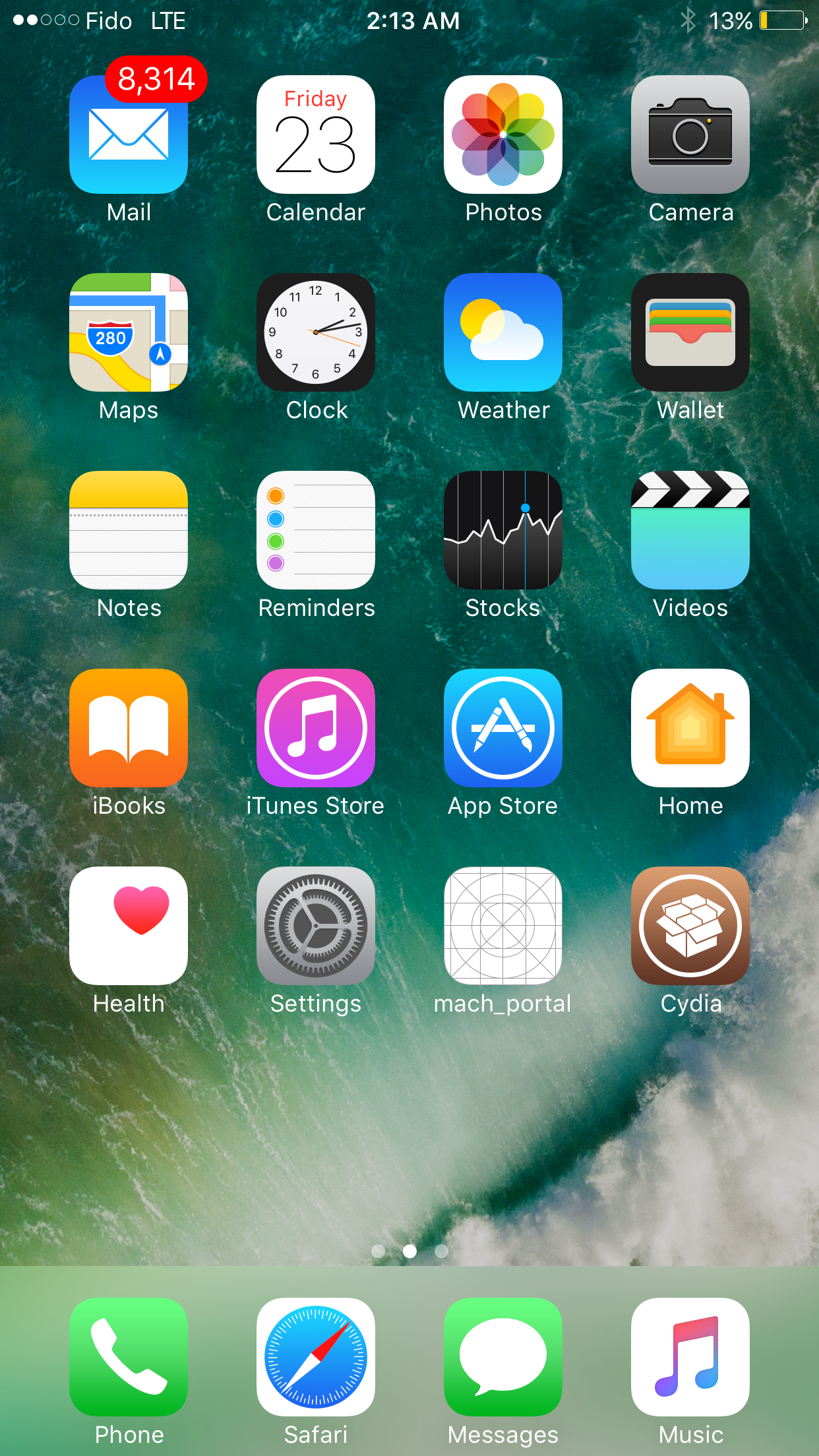The image showcases the home screen of an Apple iPhone. At the top left corner, the cellular signal strength is shown with two out of five bars, and the network provider is FIDO. The device is connected via LTE. In the top center, the time is displayed as 2:13 a.m. On the top right, the Bluetooth icon is visible along with the battery indicator, which is yellow and shows a 13% charge. 

The home screen features several app icons arranged in a grid:

- **First row:** Mail, Calendar, Photos, Camera
- **Second row:** Maps, Clock, Weather, Wallet
- **Third row:** Notes, Reminders, Stocks, Videos
- **Fourth row:** iBooks, iTunes Store, App Store, Home
- **Fifth row:** Health, Settings, Mock Portal, Cydia
- **Bottom row:** Phone, Safari (web browser), Messages, Music (iTunes)

The wallpaper in the background displays a serene waterfall with greenish-colored water, adding a picturesque touch to the home screen.